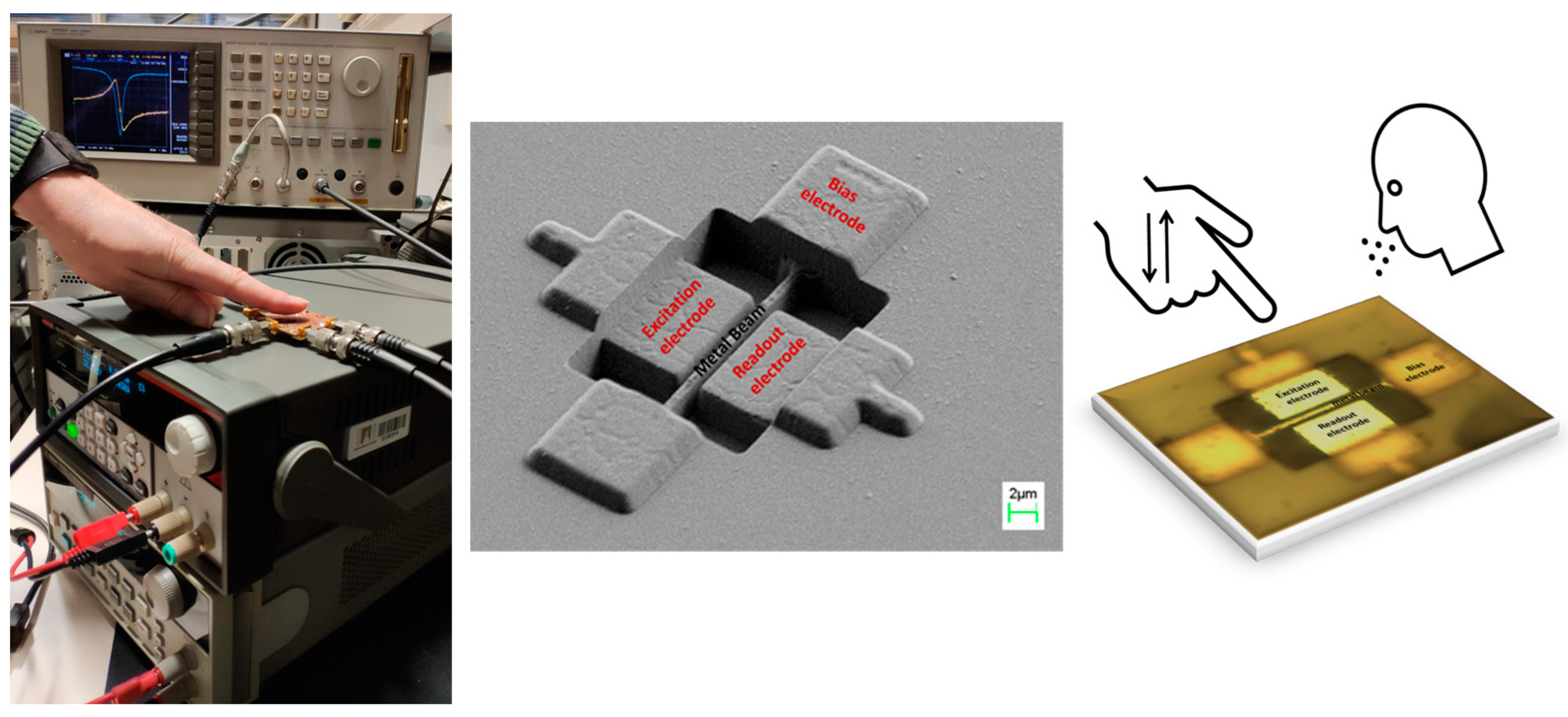The image is a triptych featuring detailed observations of electronic components. In the first photograph, a hand, partially obscured by a green and blue sweater and wearing an indeterminate wrist accessory, points at a specific section of a black electronic machine. This machine is intricate, featuring many switches, knobs, and wires, with a white medical device—likely a heart monitor—visible behind it displaying characteristic heartbeat lines. In the second image, the focus is on a gray label that reads "BING electronic," potentially indicating a section of the device seen in the first image. The label also shows elements like four quadrants with buttons. In the third image, a yellowish olive rendition of the four-quadrant chip is depicted, this time illustrated with a cartoon hand pointing towards it and a white cartoon head emitting dots from its mouth, giving the impression of speech or instruction.